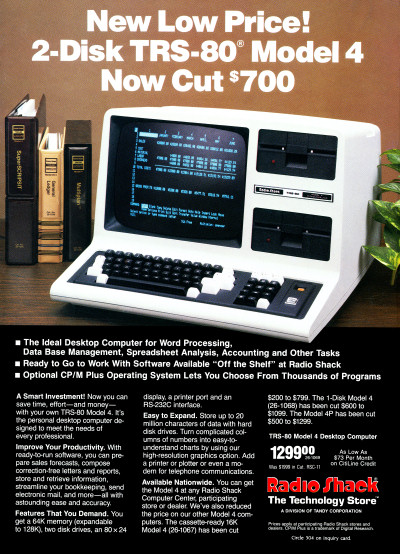This is a detailed page from a magazine advertising the Radio Shack TRS-80 Model 4 computer, an early edition targeted at general office tasks. The ad highlights "New Low Price" in bold white text, announcing a $700 price cut. The emphasized price of the computer is $1,299. The TRS-80 Model 4 features a small screen with integrated keyboard and two black floppy disk drives, built into a single white unit. The screen displays blue text and numbers, although the exact content isn't clear. To the left of the computer are some loose-leaf binders, all resting on a brown and black wood grain table. On the right edge of the image, a few leaves of an office plant are visible. 

Below the image, on a black background with white text, several key features are listed:
1. Ideal for word processing, database management, spreadsheet analysis, accounting, and other tasks.
2. Ready to go to work with software available off the shelf at Radio Shack.
3. Optional CP/M Plus operating system allows users to choose from thousands of programs.

The bottom of the ad contains three columns of text with detailed specifications and features, but the text is difficult to read. The ad concludes with the red Radio Shack logo and the slogan "The Technology Store" in white text.